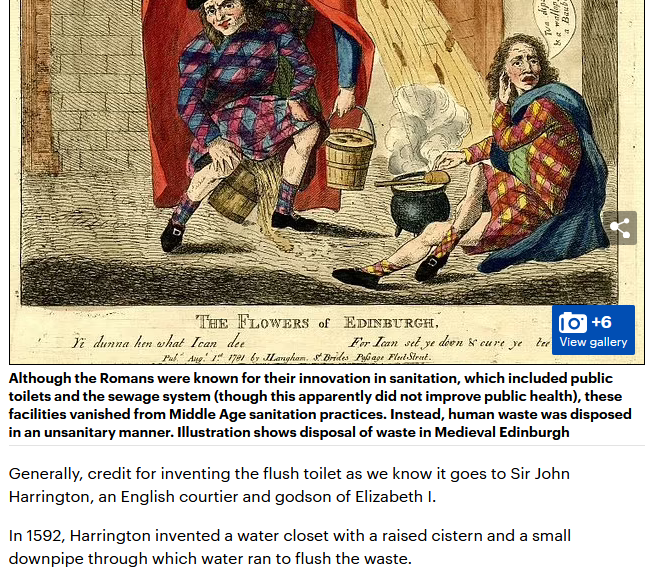The image is a detailed and colorful illustration that appears to be quite old, featuring an aged, yellowed page with a vintage font. The caption at the bottom of the image reads "The Flowers of Edinburgh." This historical illustration depicts two light-skinned individuals in a medieval setting. 

The person in the center wears a multicolored robe in shades of blue, black, and pink, with bare legs, matching socks, and black shoes adorned with silver buckles. They have a broad-brimmed hat that is mostly cut off from view and are carrying a wooden bucket. To the right, another person is seated on the ground, dressed in a plaid robe similar to the one worn by the standing figure. This individual also sports matching socks and black shoes with silver buckles, and has long blondish hair. Beside them on the ground is a black kettle, with steam or smoke rising from it, suggesting it contains a hot liquid.

Beneath the image, detailed text elaborates on historical sanitation practices, explaining that although the Romans made significant advancements with public toilets and sewage systems, these innovations did not last into the Middle Ages. In medieval Edinburgh, human waste was disposed of in an unsanitary manner, as illustrated by the scene. Additional information discusses the development of flush toilets, crediting Sir John Harrington with the invention of an early water closet in 1592.